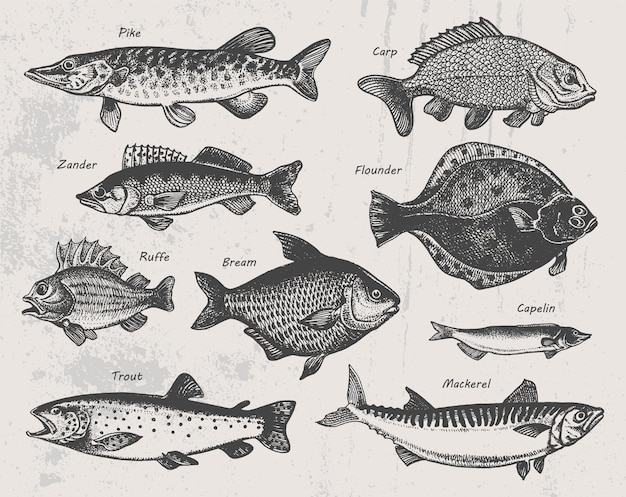This is a detailed drawing illustration of nine different fish species, arranged against a textured, light gray, khaki-colored background. The fish are depicted in black and white, with each one facing either left or right, likely for illustrative clarity. From the left to the right and down, the fish are organized as follows:

1. **Pike**: Positioned towards the top facing left.
2. **Zander**: Below the pike, also facing left.
3. **Roughfish (Ruffy)**: The smallest of the fish facing left, noted for its large, scaly dorsal fin.
4. **Trout**: Completing the left-facing sequence.
5. **Bream**: Centrally located, facing to the right, standing out as it faces a different direction.
6. **Carp**: Positioned to the right side and facing right.
7. **Flounder**: Unique for its flat body and both eyes on one side, facing right.
8. **Capelin**: The smallest fish on the right, resembling a mackerel.
9. **Mackerel**: Larger and situated below the capelin, also facing right.

The background texture and classic style lend the illustration a somewhat dated, scientific illustration feel, capturing the intricate details and subtle differences between the fish. Despite their diverse shapes and features in reality, they appear similarly sized in this drawing. The illustration lacks any additional wording other than the labels for each fish species.